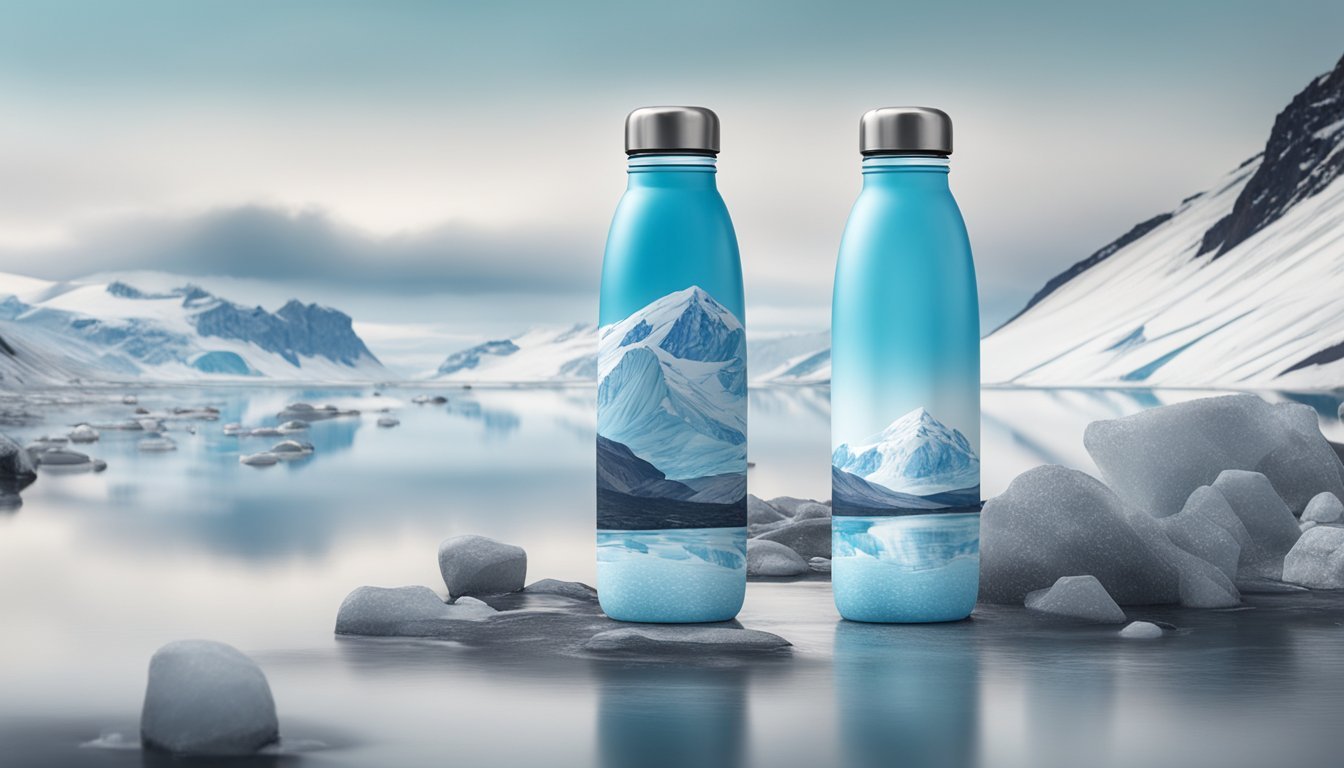In a digitally crafted Arctic or Antarctic landscape, characterized by serene, ice-blue waters and snow-capped mountains under a cloudy sky, two water bottles sit prominently in the foreground. Each bottle, adorned with vibrant, cartoonish depictions of icy mountains and water, contrasts sharply with the photorealistic yet computer-generated scenery. The bottles, featuring screw-off silver caps, have no labels or writing, emphasizing the artistic design. They rest on a surface that could be ice or a shallow rocky area surrounded by the calm, reflective water. The overall composition cleverly blends the illustrated mountainous scenes on the bottles with the snowy peaks of the background, creating a seamless, immersive visual narrative that highlights the merging of art and nature.